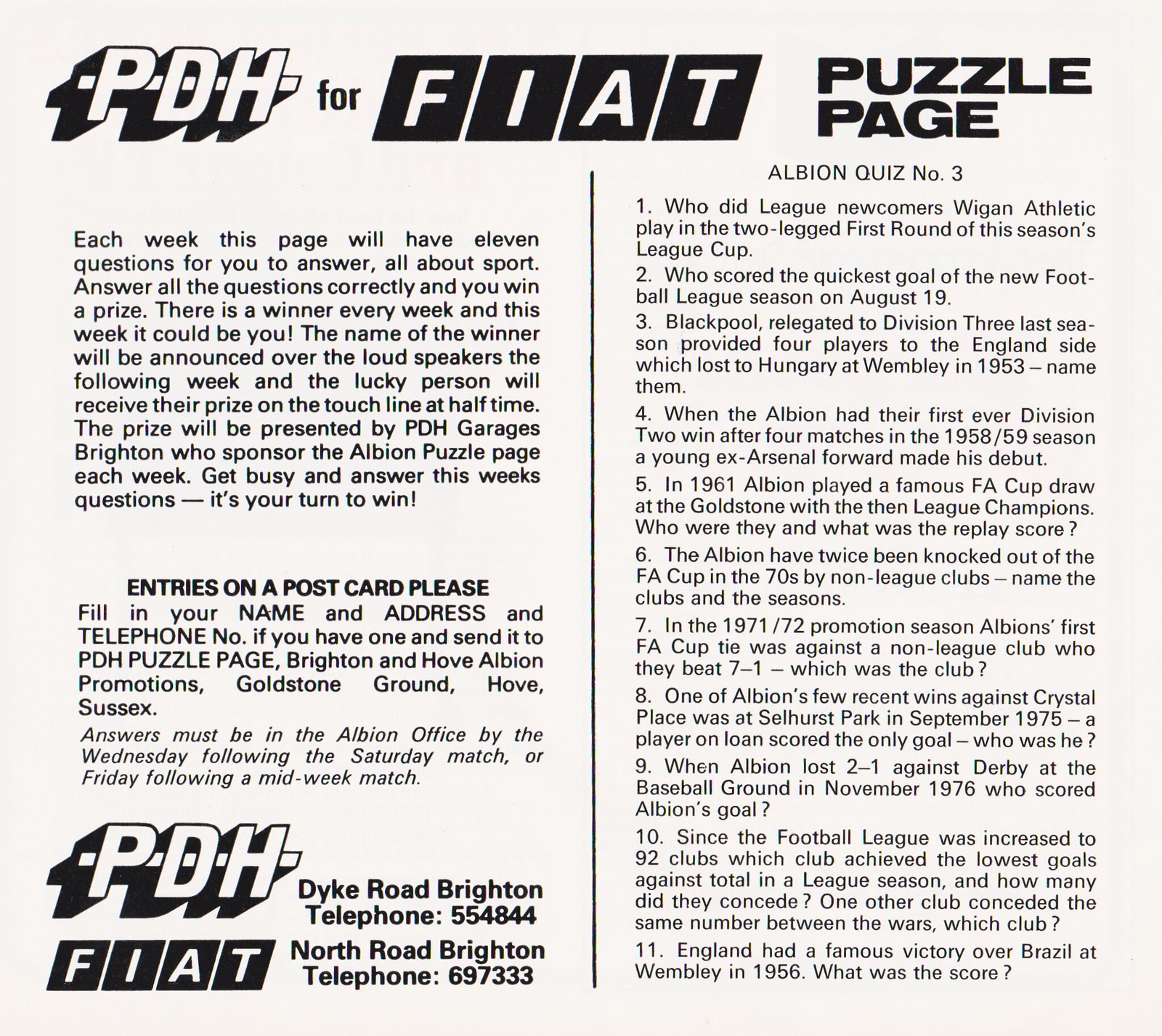This image appears to be an excerpt from a vintage magazine or newspaper, featuring a section titled "P.D.H. for Fiat Puzzle Page" in 3D white font outlined in black. Below that, in bold black text, it states "Puzzle Page." The left column introduces the quiz, mentioning that "Each week this page will have 11 questions for you to answer, all about sport. Answer all the questions correctly and you win a prize. There's a winner every week and this week it could be you." It further explains that the winner's name will be announced over the loudspeakers the following week, with the prize, presented by P.D.H. Garage's Brighton, awarded on the touchline at halftime.

Participants are instructed to send their answers on a postcard, including their name, address, and telephone number, to "P.D.H. Puzzle Page, Brighton and Hove Albion Promotions, Goldstone Ground, Hove, Sussex." Answers must reach the Albion office by the Wednesday after a Saturday match or the Friday following a midweek match. The left column also features the P.D.H. Fiat logo, providing contact details for their Dyke Road and North Road locations in Brighton.

The right column is titled "Albion Quiz Number 3," containing 11 sports-related trivia questions. Example questions include, "Who did league newcomers Wigan Athletic play in the two-legged first round of this season's League Cup?" and "Who scored the quickest goal of the new football league season on August 19?" Other questions cover historical events and achievements in football, such as notable games, player debuts, and club statistics.

The detailed description effectively combines the shared and repeated elements from all three original captions to create a comprehensive and cohesive summary of the image.